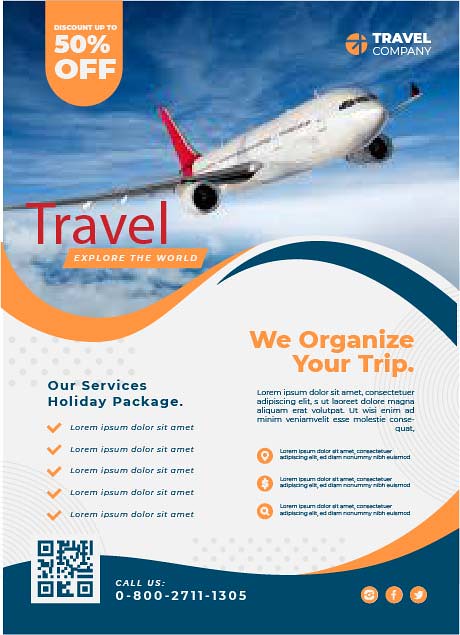This vibrant advertisement poster is designed to promote a travel service. Dominating the visual at the top, a white airplane with a red tail soars through a blue sky adorned with white clouds. To the top right of the poster, "Travel Company" is prominently displayed, while the top left corner features an orange dot announcing a discount of up to 50% off. Below the airplane, bold red text reads "Travel," followed by the phrase "Explore the World" in orange with white letters.

The middle portion of the advertisement transitions to a white background showcasing additional service details in a non-English language, though key phrases such as "Our Service Package" and "We organize your trip" are visible. Towards the bottom left, a QR code is provided, accompanied by the contact number 0800-2711-1305. Adjacent to the QR code are orange social media icons for Instagram, Facebook, and Twitter, featuring white logos. The bottom section of the ad is a striking blue, tying the design elements together cohesively.